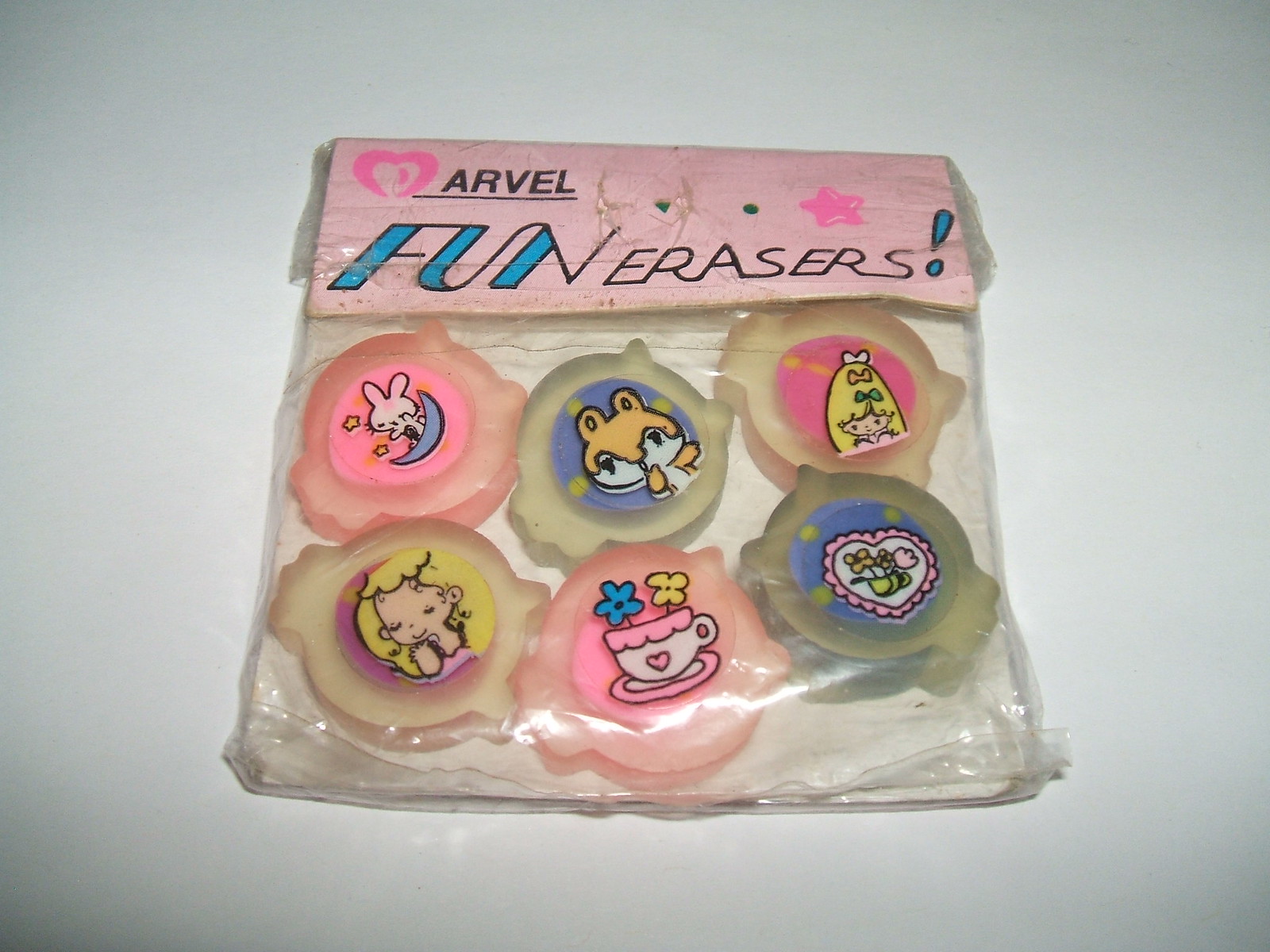The image features a slightly worn, unopened package of "Arvel Fun Erasers," set against a white background. The clear plastic packaging showcases six circular erasers, each adorned with unique, colorful illustrations: a bunny sitting on a moon, a girl with bows in her hair, a teacup with flowers, a hamster (possibly a chipmunk), a blonde girl waving, and a heart doily with flowers. The pink top label of the package appears to be hand-designed, with "Arvel" written in blue letters followed by a pink heart and "Fun Erasers" in an exclamation-filled script, giving it a homemade, nostalgic feel. This resembles a product that might be found at a dollar store.